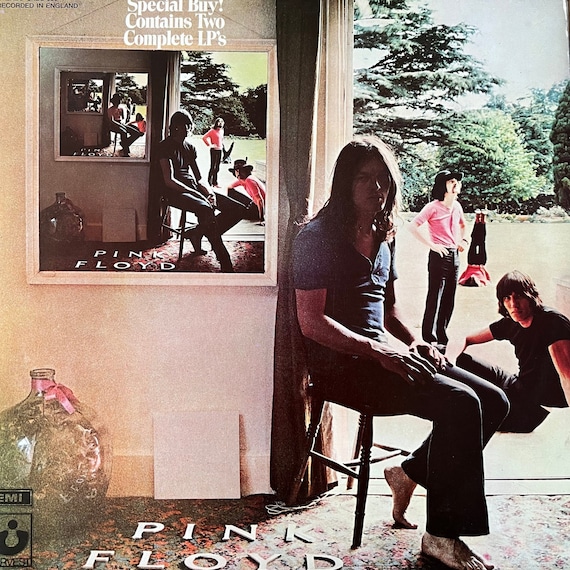This album cover for Pink Floyd, "Recorded in England," is an intriguing composition featuring a multi-layered scene. At the top left corner, it prominently mentions "Special Buy Contains 2 Complete LPs." The cover is dominated by a man with long, dark hair, wearing a blue short-sleeved shirt and jeans, sitting barefoot on a stool. His face is in the shadows, making his hair appear almost black. He is seated inside a doorway, against a backdrop of an elaborate, colorful rug in shades of pink, brown, and blue, with "Pink Floyd" spelled out in white letters on the floor. 

To his left, a mirror reflects the same scene, slightly altered, where members of the band are arranged differently. Outside the doorway, a man in black attire sits on the steps and another stands nearby. In the background, another person lies on the concrete with legs raised, while one more figure can be seen seated. The entire image, both in the mirror and outside, captures a sense of perpetual reflection, echoing the intricate and surreal nature of Pink Floyd's music.